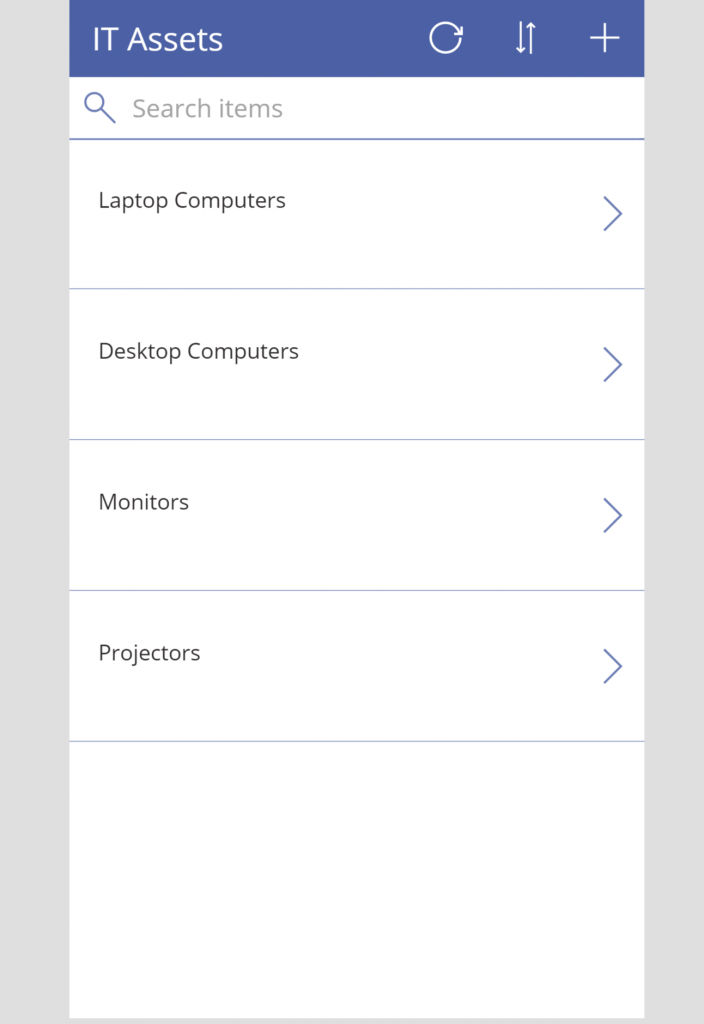An image depicts a minimalistic interface for managing IT assets, likely designed for an office environment. The clean white background enhances the sparse layout, which is delineated by clear spacing between elements. At the top, a header reads "IT Assets." Directly below are four categorized items: Laptop Computers, Desktop Computers, Monitors, and Projectors. A search bar, labeled "Search Items" in dim gray text hinting for user interaction, features a small magnifying glass icon as a visual cue.

Additional interface elements include a refresh button and an adjacent button with an arrow pointing up and an arrow pointing down, potentially indicating upload or download functions. A plus button is also present, possibly for adding new items to the list. The overall aesthetic is utilitarian and straightforward, underscoring its intended use in a business setting rather than for general consumers. The limited scope of items suggests that this tool is specifically tailored for managing essential IT equipment.